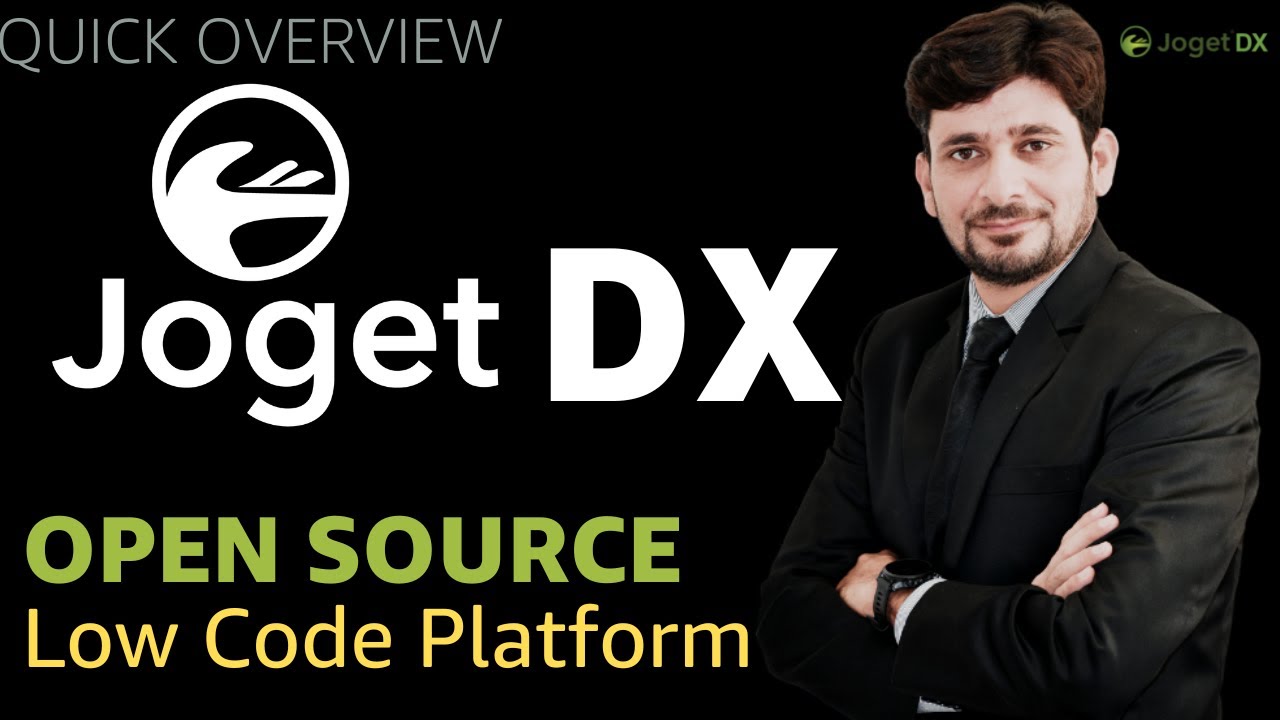A detailed internet advertisement screenshot features a prominent black background. In the center, large white text reads "JogetDX," complemented by a round icon above that resembles a shovel pointing left with grass sprouting from it. The top left corner is marked with the phrase "Quick Overview" in a light white font. Positioned towards the bottom, in large light green text, is the phrase "Open Source," followed by "Low Code Platform" in slightly smaller yellow font beneath it. The JogetDX logo, located on the right, is displayed in light green for "Joget" and a brighter green for "DX," accompanied by the same round icon.

To the right of center, a man is depicted in a suit. He appears to be of Persian or Middle Eastern descent, with light-ish skin. His dark brown hair, which includes reddish highlights, is parted to the left side of the photo. He sports a goatee that seamlessly blends into sideburns reaching his hairline. The man is clad in a black suit, a white collared shirt, a long black tie, and a wristwatch on his left wrist. Although his suit looks refined, its slightly wrinkled appearance suggests tension or movement in his crossed-arm stance.